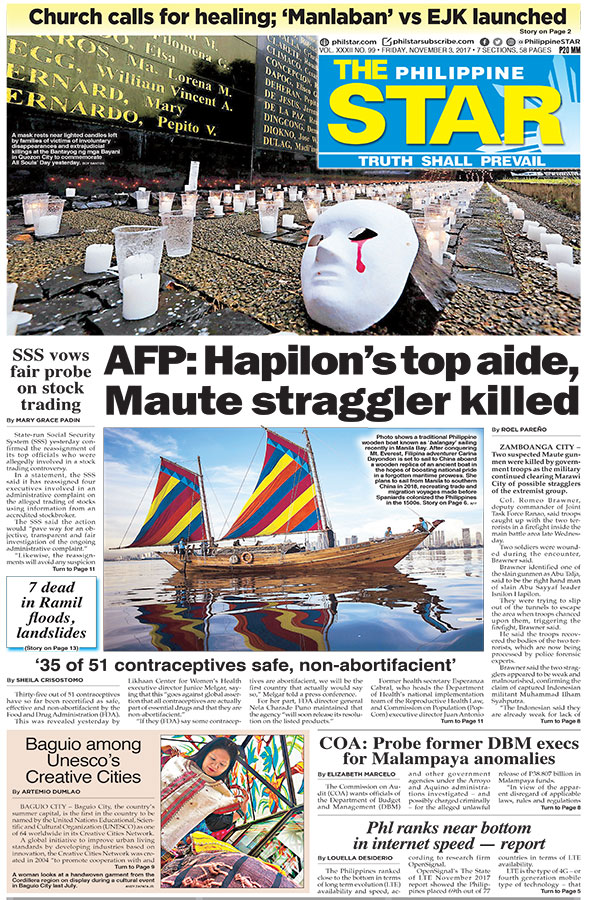**Descriptive Caption:**

This image is a detailed screenshot of a newspaper page. At the top, a prominent yellow bar features the headline, "Church Calls for Healing; 'Man Laban vs BJK Launched'." Below this title, there are small, barely legible icons and communication symbols. The centerpiece of the header includes a large yellow rectangular box with "The Star" prominently displayed, accompanied by the phrase "Philippine" in white text above it and "Truth Shall Prevail" in white beneath.

A large photograph dominates about a third of the page, depicting a white mask with a red tear streaming from one eye. The mask is set on a sidewalk, surrounded by approximately eight rows of at least 30 white candles, some of which are placed in cups. Adjacent to this solemn setup is a black memorial wall inscribed with white names.

Beneath the photograph, the headline reads: "AFP: Hapilon's Top Aid Maute Mount Straggler Killed." To the left, a sidebar headline states, "SSS Vows Fair Probe on Stock Trading." An adjacent article begins with, "Seven Dead in Ramil Floods, Landslides."

In the lower middle section of the page, another photograph depicts a wooden boat adorned with two colorful flags, reflecting in the water with a city skyline in the background. The accompanying article is titled, "35 of 51 Contraceptives Safe, Non-Abortifacient."

On the right-hand side of the page, although the exact text of one article is difficult to discern, the bottom section features the headline, "Baguio Among UNESCO's Creative Cities," next to a photograph of a woman holding up a blouse as if shopping. Two additional articles complete the layout on the right side of the page.